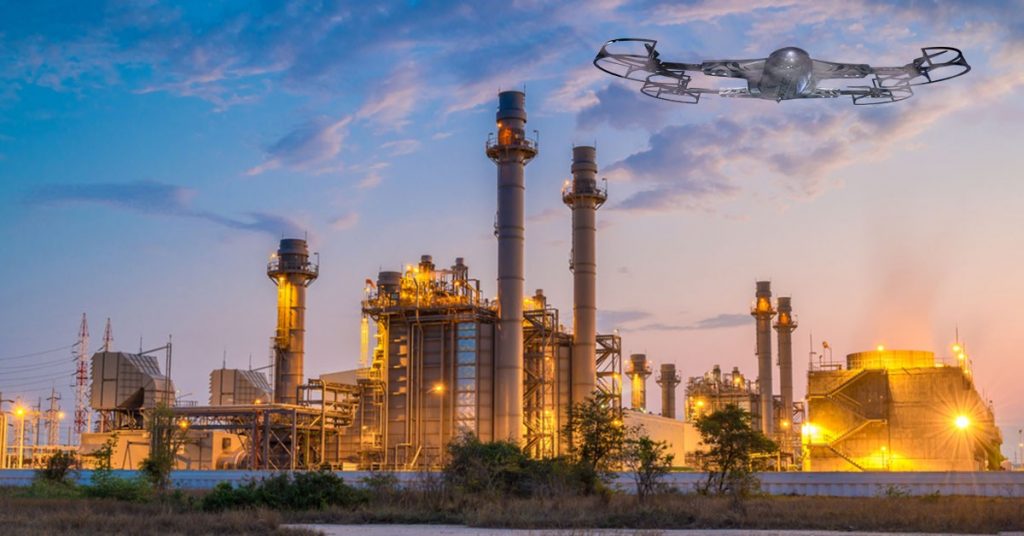The photograph depicts a sprawling industrial plant set against a landscape that includes grassy areas and some trees in the foreground. The scene is viewed from across a river, with natural shrubbery and a white border wall marking the perimeter. The sky transitions from a deep blue in the top left to a pinkish hue towards the bottom right, suggesting early evening or sunset. Various smoke-stacks pepper the site, emitting a hazy, smoky atmosphere that lends a slightly obscured view of the complex. The factory features a mix of different-shaped buildings of varied heights, illuminated by bright, yellowish, and gold-hued lights. Tall cylindrical towers, which look like watchtowers, surround the buildings, seemingly for protection. Adorning the industrial labyrinth is a drone, gray in color and the size comparable to an airplane, hovering in the upper right-hand corner with four propellers. This drone, with its distinct appearance, adds a futuristic element to the otherwise industrial scene. Power lines crisscross the plant, amplifying the very industrial aesthetic of the whole setup.